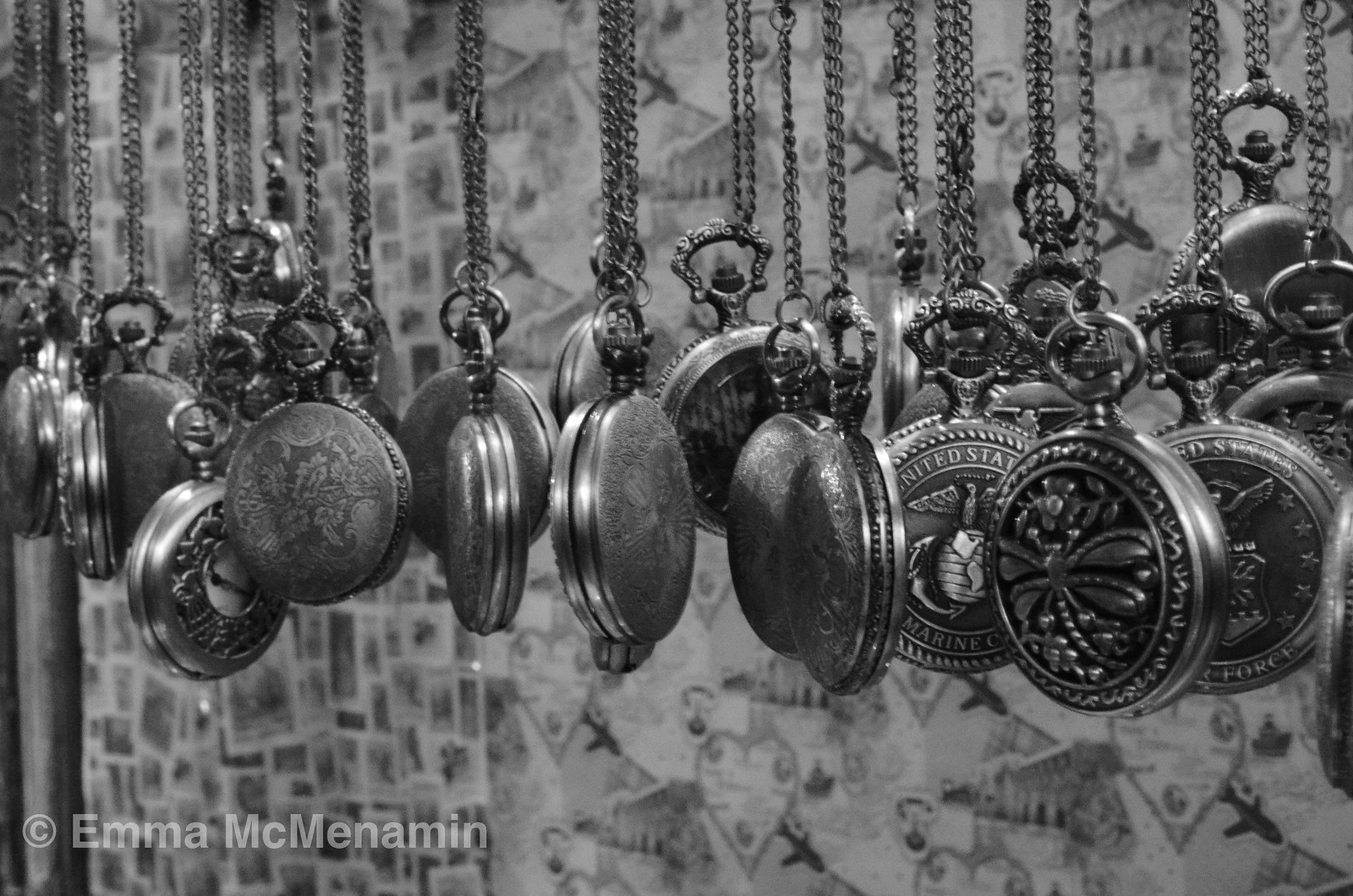This black and white photograph showcases an array of hanging pocket watches, each suspended by fine chains that disappear out of the frame. There are at least sixteen pocket watches, all round and roughly the same size but adorned with diverse, intricate designs. Some display crests and one notably features a dragonfly, while others bear flowery, ornate patterns. A few watches in the middle exhibit lighter, delicate designs, while those towards the edges have more robust, carved embellishments. Notable among the decorations are a couple of watches with United States Marine Corps insignias, hinting at a possible military theme.

The watches hang against a backdrop that is hard to clearly define; it might be a patterned curtain, collage of photographs, or newspapers. Towards the right side of the background, small planes can be seen decorating the tapestry-like surface. In the bottom left corner, a translucent gray copyright symbol reads "Emma McMenamin," subtly overlaying the image without detracting from the detailed display of the pocket watches.